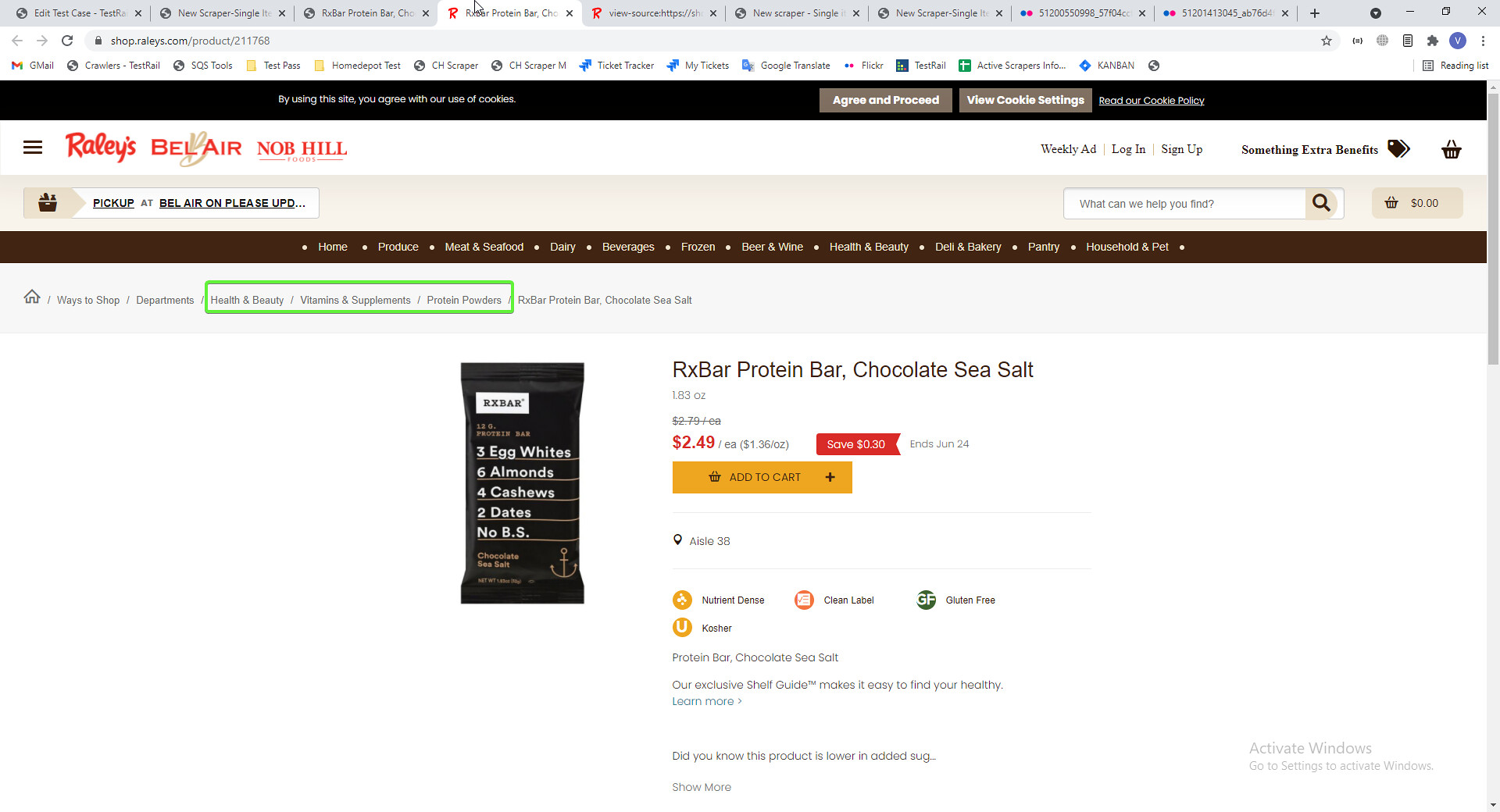The image is a color screenshot from a website called Rallies, Mellor, and Nob Hill, showcasing an RX Bar Protein Bar in the Chocolate Sea Salt flavor. The bar's packaging is black and prominently displays "3 egg whites, 6 almonds, 4 cashews, 2 dates, no BS." The product is originally priced at $2.79 each but is currently on sale for $2.49 each, equivalent to $1.36 per ounce, offering a savings of $0.30. This sale ends on June 24th. The website's interface shows various browser tabs and bookmarks, indicating it is a platform that offers a variety of treats, as well as beer and other beverages, suggesting it might be an online grocery store.